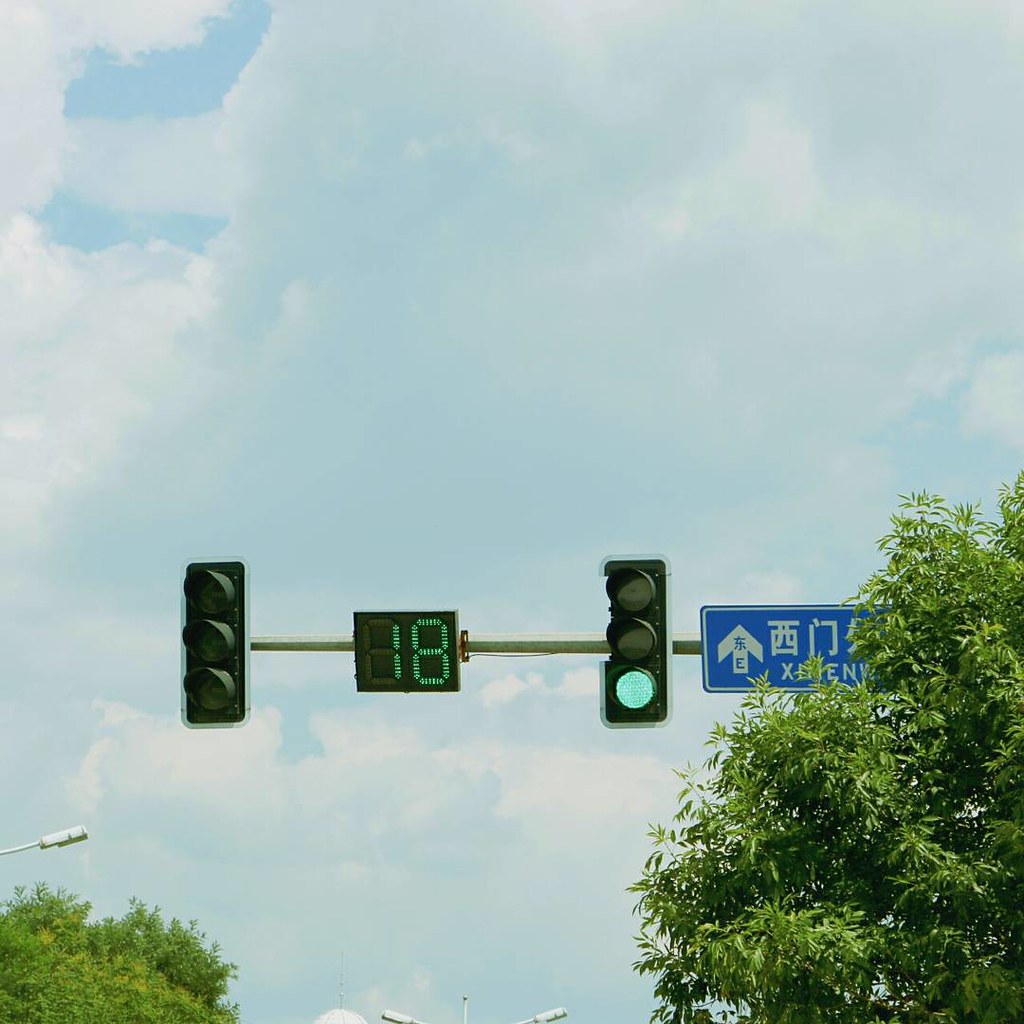The photograph captures a street scene featuring a traffic light setup against a light blue sky adorned with fluffy white clouds. Centered on a horizontal pole are two traffic lights. The one on the left has all its lights off, exhibiting its typical red, yellow, and green circles. In the middle, there is an illuminated numerical display showing the number 18 in green. The right traffic light has its bottom green light on. To the right of these is a rectangular blue sign with white text and an upward-pointing arrow, though much of it is obscured by a large green tree. The text on the sign appears to be in Japanese. Additionally, near the bottom of the image, parts of green trees and three white overhead lights are visible.